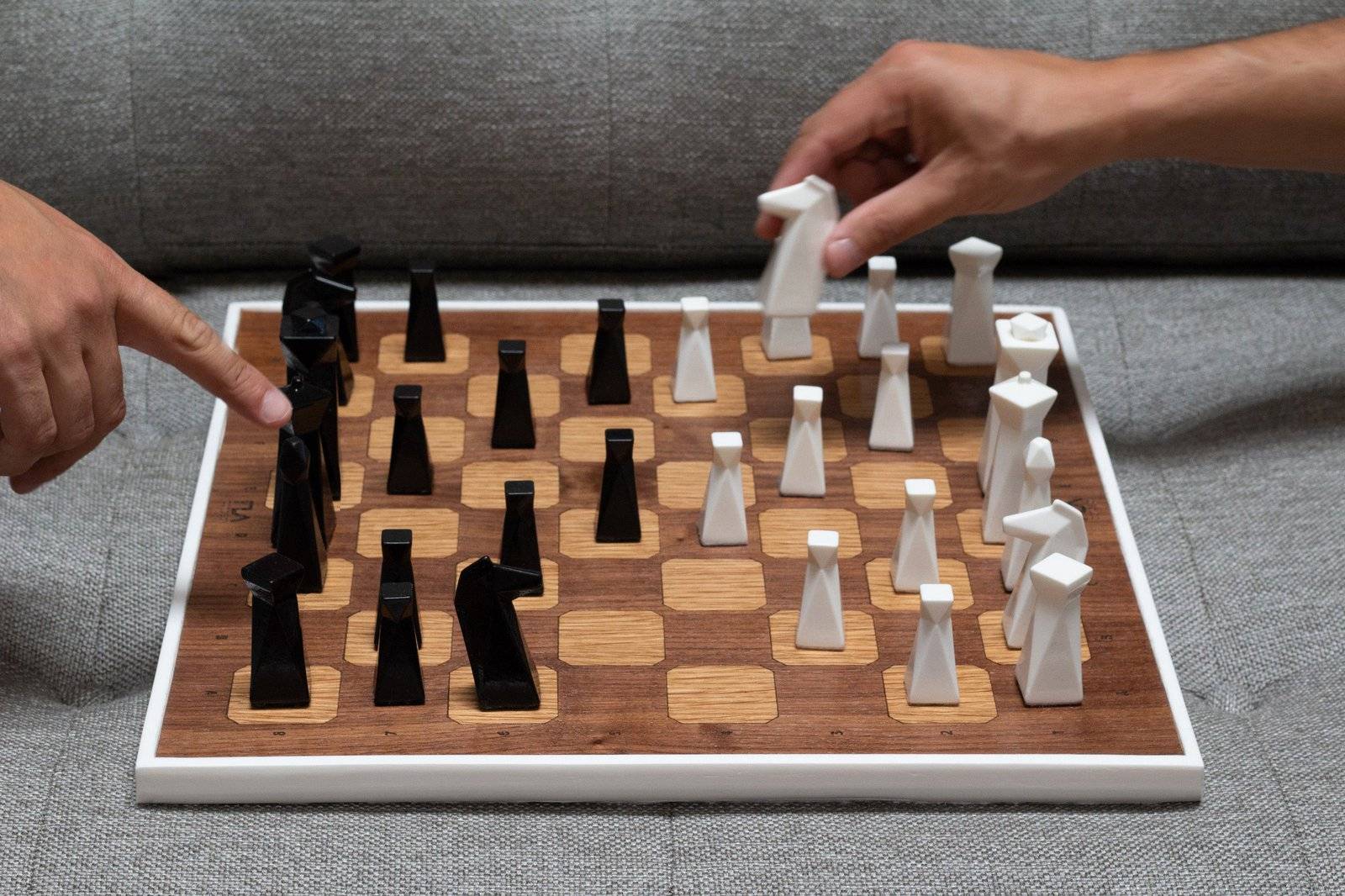In this detailed image, a wooden chessboard with dark and light wood squares sits on a grey fabric couch. The board is bordered in white and features onyx pieces on the left and ivory pieces on the right. The game appears to be in progress, as some pawns have already moved forward. On the left side of the image, a man's right hand is visible from mid-hand to fingers, with his index finger pointing at his row of black chess pieces, possibly indicating a move or suggesting a strategy. On the right side, another hand, visible from mid-forearm to fingers, grips the largest piece on the board, an ivory knight, between the index finger and thumb, poised to make a move. The scene suggests a moment of instruction or decision in the midst of an ongoing chess match.